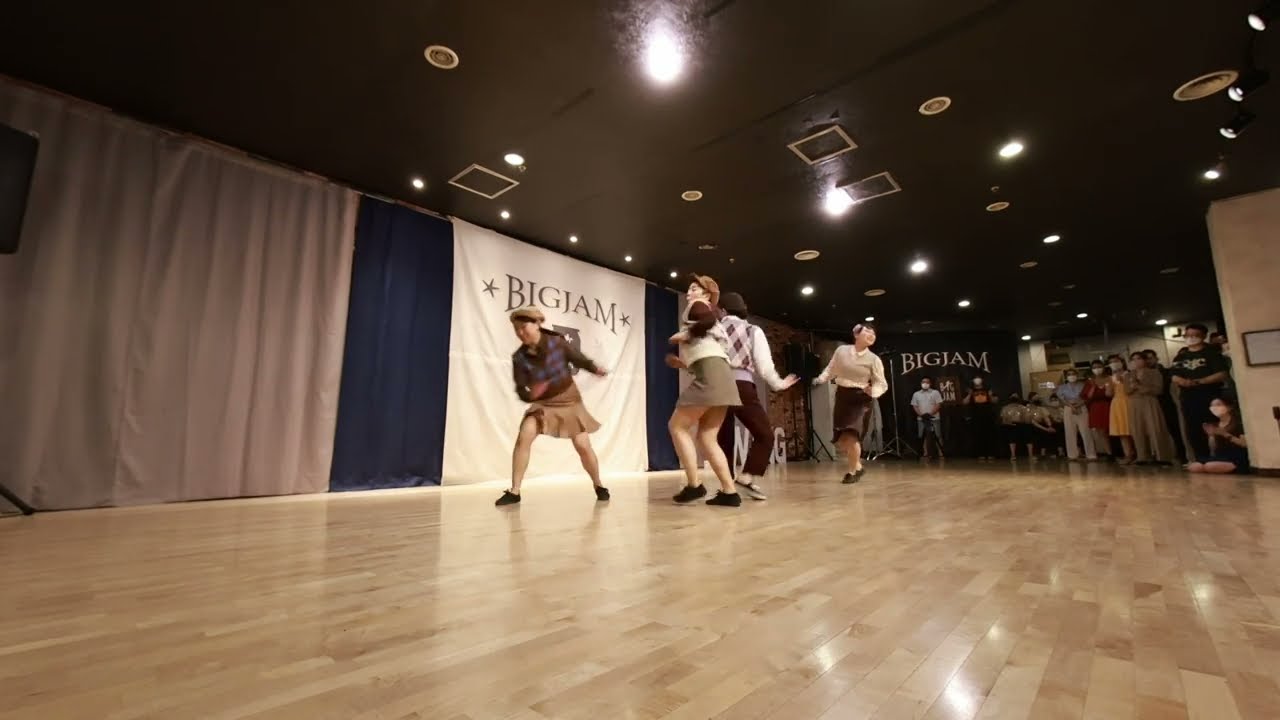The image captures a vibrant dance performance set on a shiny wooden floor made of light tan, rectangular wood paneling. At the forefront, there are four individuals, three of whom are women wearing 1950s-style dresses: two in light tan skirts paired with plaid shirts, and one in a deep brown dress with a light tan shirt. The fourth individual, likely a man, is dressed in brown slacks, a white shirt, a sleeveless vest, and a hat. All of them are also wearing hats, adding a cute touch to their ensemble. The backdrop consists of a grey curtain followed by a blue one, from which a large white sheet with the words "Big Jam" in khaki-colored writing hangs prominently. A similar "Big Jam" sign hangs in another part of the venue.

The setting features a black ceiling adorned with multiple light fixtures and ventilation. In the background, a sizable crowd watches attentively; most of the spectators are wearing white face masks, possibly due to COVID-19 precautions. Despite the masks, there's a noticeable sense of joy and excitement, with at least two visible smiles hinting at the fun atmosphere of the event. The overall scene resembles a lively dance competition, capturing both the nostalgic costumes and the upbeat spirit of the moment.